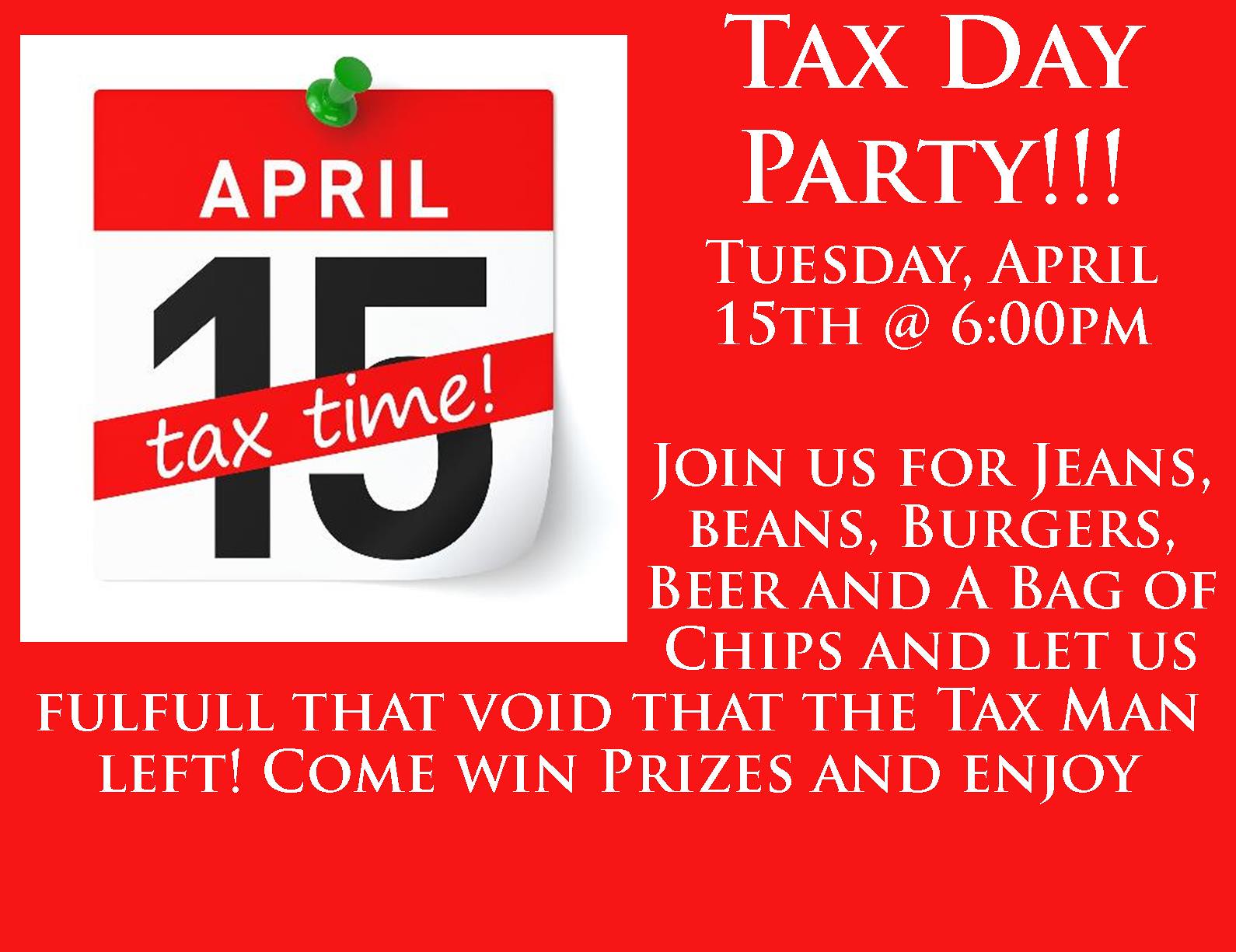This is an advertisement flyer for a Tax Day Party. The flyer has a bold red background with predominantly white and black text. At the top right corner, large white letters announce "Tax Day Party" followed by three exclamation points. Directly beneath this headline, the date and time are provided in smaller print, stating, "Tuesday, April 15th at 6 p.m."

On the upper left corner of the flyer, there is a visual of a calendar page pinned with a green push pin. The calendar page has a red banner at the top that says "April" in white letters, and below that, a large black "15" marking the date. A red banner across the "15" proclaims "Tax Time!" with an exclamation point. 

Towards the bottom of the flyer, an invitation encourages people to "Join us for jeans, beans, burgers, beer, and a bag of chips," adding, "let us fulfill that void that the taxman left!" This is followed by, "Come win prizes and enjoy." This text, like the rest, is in white letters on a red background. Aside from the green pin, the flyer features text and designs only in red, white, and black.